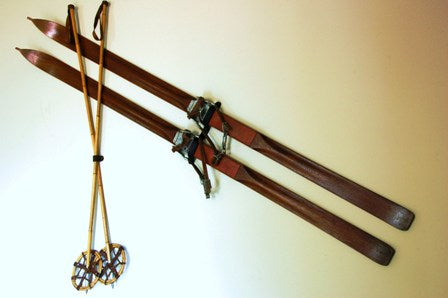This image features a rustic display of vintage ski equipment mounted on a white-beige, well-lit wall. Prominent in the center are two dark brown wooden skis with slightly lighter brown foot fastening areas highlighted by black straps. Arranged diagonally, the skis stretch from the bottom right to the top left, where their pointed tips converge. Above the skis, two light brown ski poles crisscross, their straps designed to secure the skier's grip, and round bottoms equipped with circular netting to prevent sinking into the snow. The scene is accentuated by muted brown tones, providing a nostalgic and timeless ambiance.